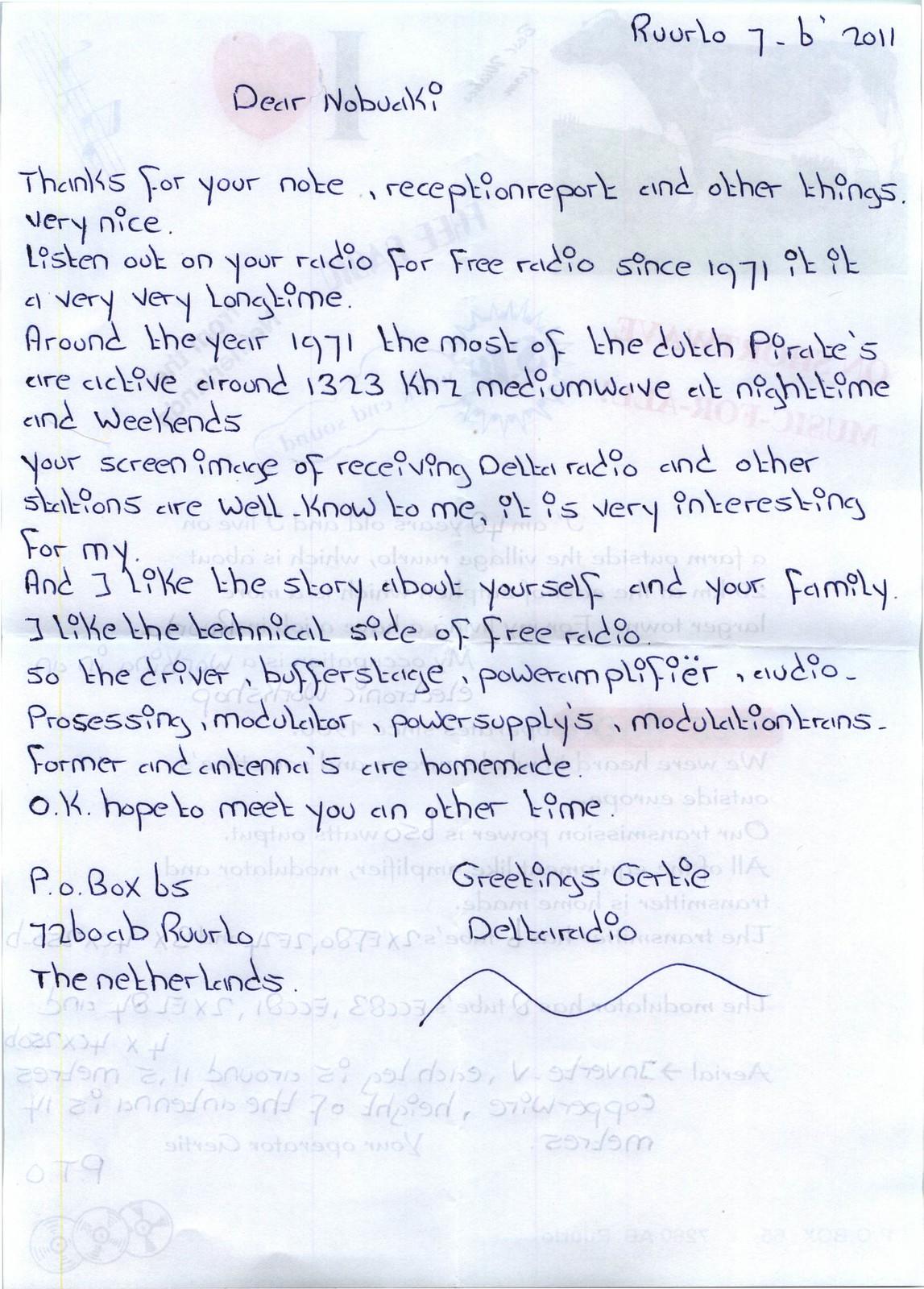The image depicts a white piece of paper with a handwritten note in blue ink. The note, addressed to Nobuaki, expresses gratitude for a previous note, mentioning a reception report and more. The writer reminisces about free radio since 1971, highlighting that during that time Dutch pirates were notably active around 1323 kHz medium wave, particularly at night and on weekends. They acknowledge the recipient's screen image of Delta Radio and other stations and show interest in the personal story about Nobuaki's family. The writer shares an appreciation for the benefits of free radio, noting that various components including the driver, buffer stage, power amplifier, audio processing, modulator, power supplies, modulations former, and antennas are homemade. The note is signed off with "Greetings, Gertie," and includes a P.O. Box address from the Netherlands. The paper appears to be partially translucent, as there might be sketches, a heart, and additional writing visible from the other side. At the top right, there is a marking that reads "Rollo 7.B 2011."